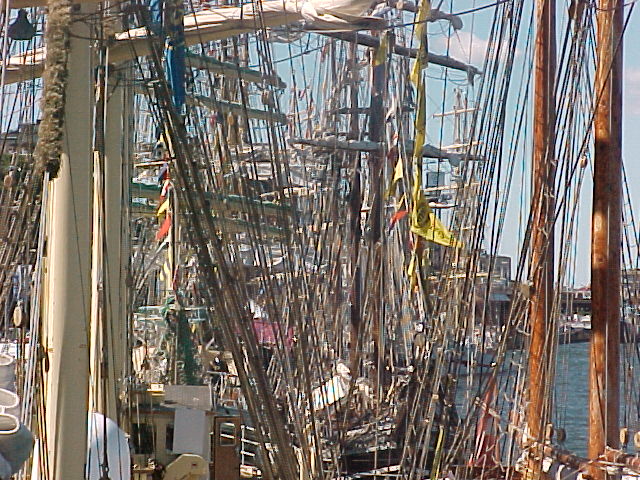An outdoor photograph captures a busy scene likely taken in a marina on a sunny day, under a light blue sky with a scattered cloud or two. Dominating the foreground are numerous masts, rigging, and lines creating an intricate jumble of cables, ropes, and poles. The masts vary in material, with some appearing as wooden and others, possibly from a separate ship to the left, made of metal. A large sailboat with several masts is seen, some adorned with red, white, and yellow flags waiting to be raised. The sails are not unfurled, but rolled up and tied horizontally. Behind this sailing vessel, blue water is visible, suggesting the presence of a secondary boat as evidenced by additional masts seen through the maze of lines. The photograph seems to be taken from the deck of another ship, providing a complex and layered maritime vista.